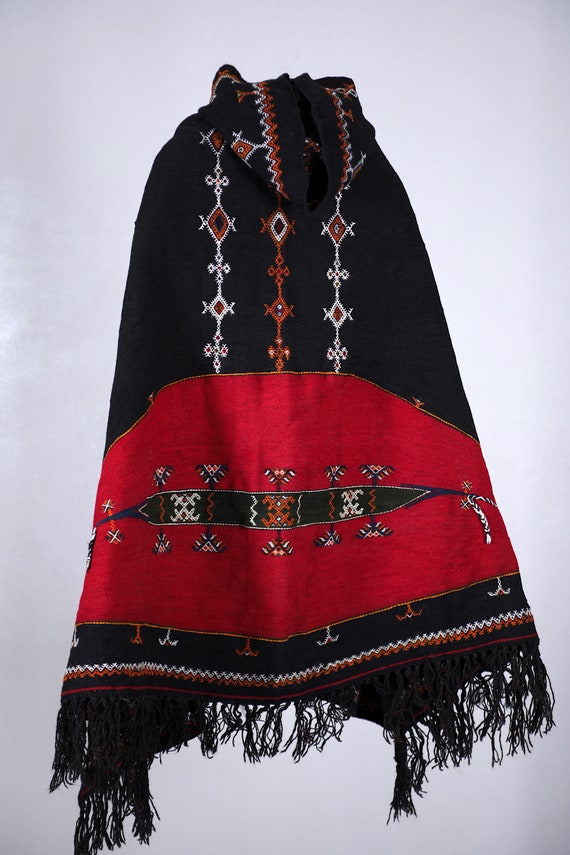This image showcases a vintage Moroccan burness, which resembles a cross between a cape and a poncho. It features a vibrant design predominantly in black and red, interspersed with intricate white and orange symbolism. The hood, located at the top, is accented with a white and orange trim against a black background. Below the hood, the cape displays a sequence of diamond shapes in white and orange, transitioning to a wide red section adorned with additional white and orange patterns. A distinctive zigzag design marks the boundary between the red section and the lower part of the cape, which is black with fringes along the hem. The burness is photographed alone, possibly for representation or sale, and is presented in a manner that highlights its detailed and cultural craftsmanship.